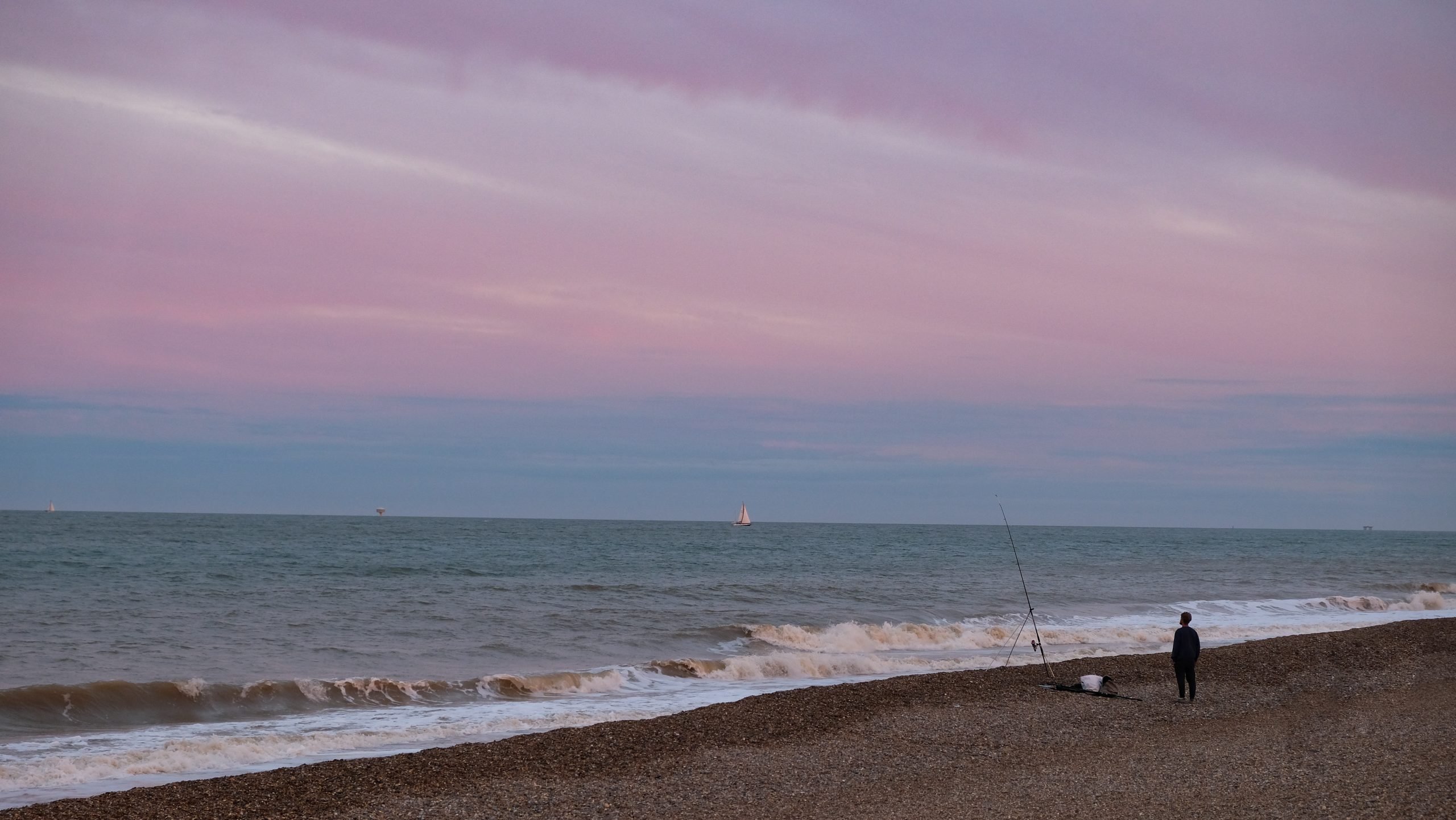The image depicts a serene and expansive beachfront vista captured just as the day ends, featuring a tranquil mix of nature's elements. Dominating the foreground, the broad, dark sand wedge extends towards the cold, blue-gray ocean. Waves crash gently along the shore, creating a delicate white froth that edges the water's boundary. To the right, a solitary figure, possibly male, stands silhouetted against the horizon, appearing small within the vast landscape. This individual seems to be alone, attempting to fish, with a fishing pole set up beside them. At their feet lies a white bucket or container accompanied by a long, black reel or object. Further into the scene, a very small white sailboat can be seen drifting in the distant water. The horizon is flat and calm, leading up to a sky painted in beautiful shades of deep somber pinkish-lilac to soft blue, mixed together in a gradient effect indicative of twilight. The entire scene exudes a peaceful atmosphere, framed by nature's calming hues and the solitary, quiet endeavor of the fisherman.